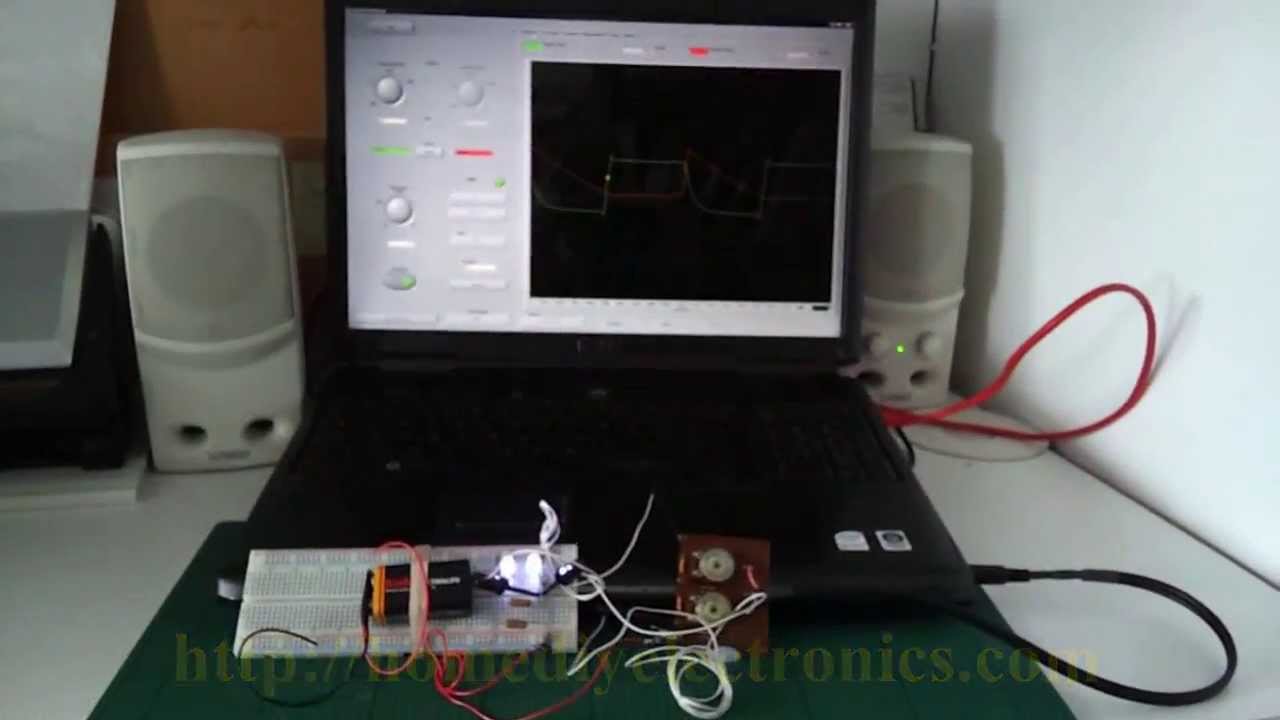The image depicts a black laptop running a diagnostic tool, prominently displaying green, yellow, and blue square waveforms on a black screen. The screen also features a distinctive yellow dot. To the left of these waveforms, there is a digital control panel with various buttons: two round buttons for scrolling right and left, a red button on the right, a green button on the left, a circular dial below these buttons, and two rectangular buttons underneath it. At the bottom is a green oblong button. Two cables, one red and one black, are connected to the laptop, with the red cable emerging from the back right and the black cable from the front right. The laptop, placed on a gray pad, is flanked by speakers on either side—one of which has a green light indicating it is powered on. The entire setup, including a circuit board connected to a nine-volt battery and possibly a cassette player, is on a white desk near a white wall on the right-hand side.